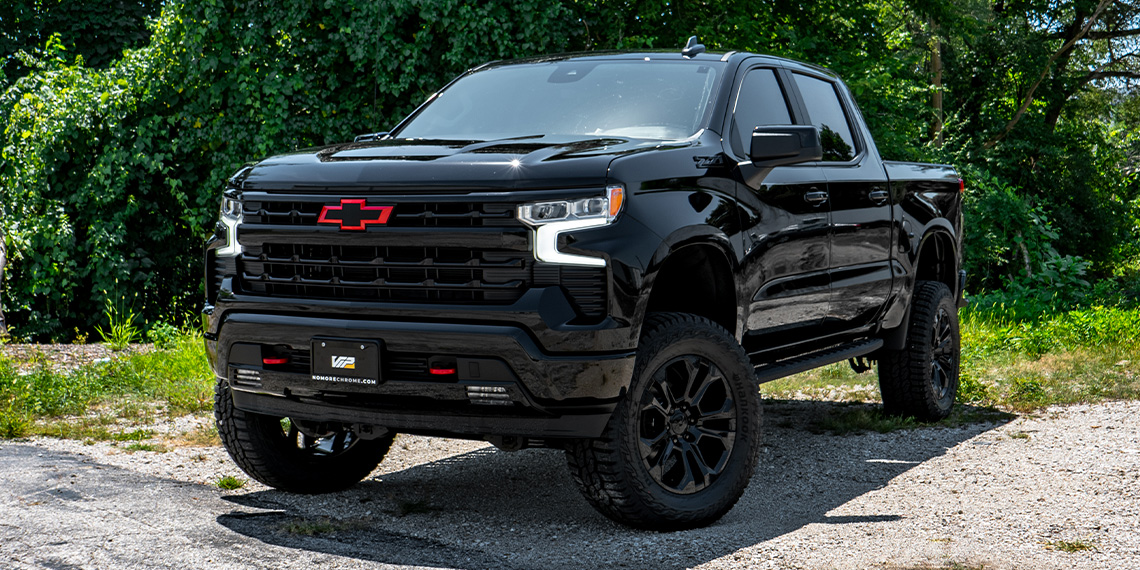This outdoor photograph captures a black Chevy pickup truck positioned at an angle, showcasing both the front and the driver's side. The truck, equipped with black rims and heavily tinted windows, sits on gravel in a sunlit area. Notably, the grille prominently features a bright red Chevrolet emblem. Below the headlights on each side, there are white square C-shaped objects. The background is filled with green shrubbery, grass, and some trees, creating a wooded setting. The truck, which has an open bed with nothing inside, casts a shadow on the ground, and there is a dot-com sticker on the bumper that is difficult to read. The front wheels are slightly tilted to the left.